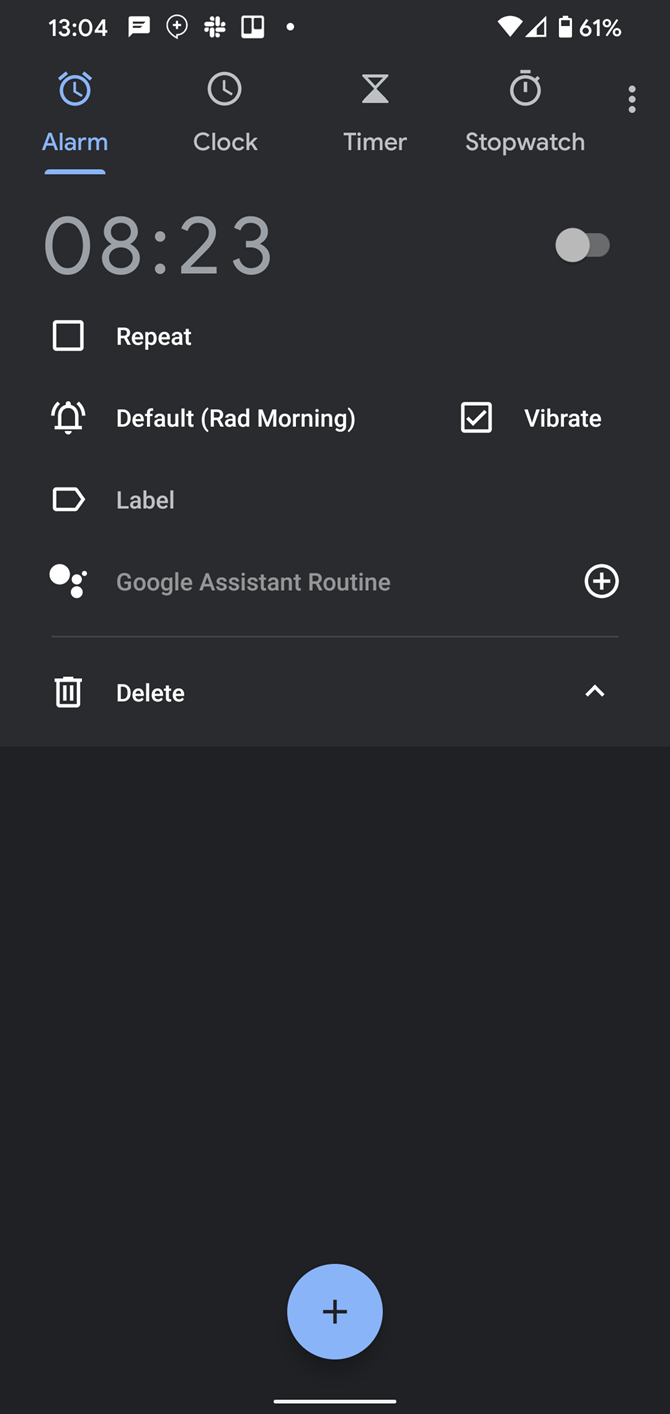A screenshot of a smartphone interface featuring various icons and notifications. At the top, the time is displayed as 13:04, alongside a "message" icon, a "plus" sign enclosed in a circle, and a "clover" symbol. Below are icons including a "box with a line in the middle", a "dot", "Wi-Fi", and "data" signals. The battery indicator shows 61%, and an "alarm" symbol is present.

The main screen displays a deep blue background with multiple utilities: a clock showing options for timer, stopwatch, and three gray dots. The number 823 is visible next to a toggle switch, and a white square is shown, likely indicating a selection option. The display includes repetitive options labeled "default," an active "bell" symbol, lines framing either side, and a text reading "Rad Morning." There is a vibrate feature enabled, indicated by a check mark. 

Further down, the words "Google Assistant Routine" are displayed next to another "plus" sign in a circle, and a "delete" icon represented by a trash can. Finally, an up arrow is visible, along with a blue circle containing a plus sign, accompanied by a white line at its bottom.